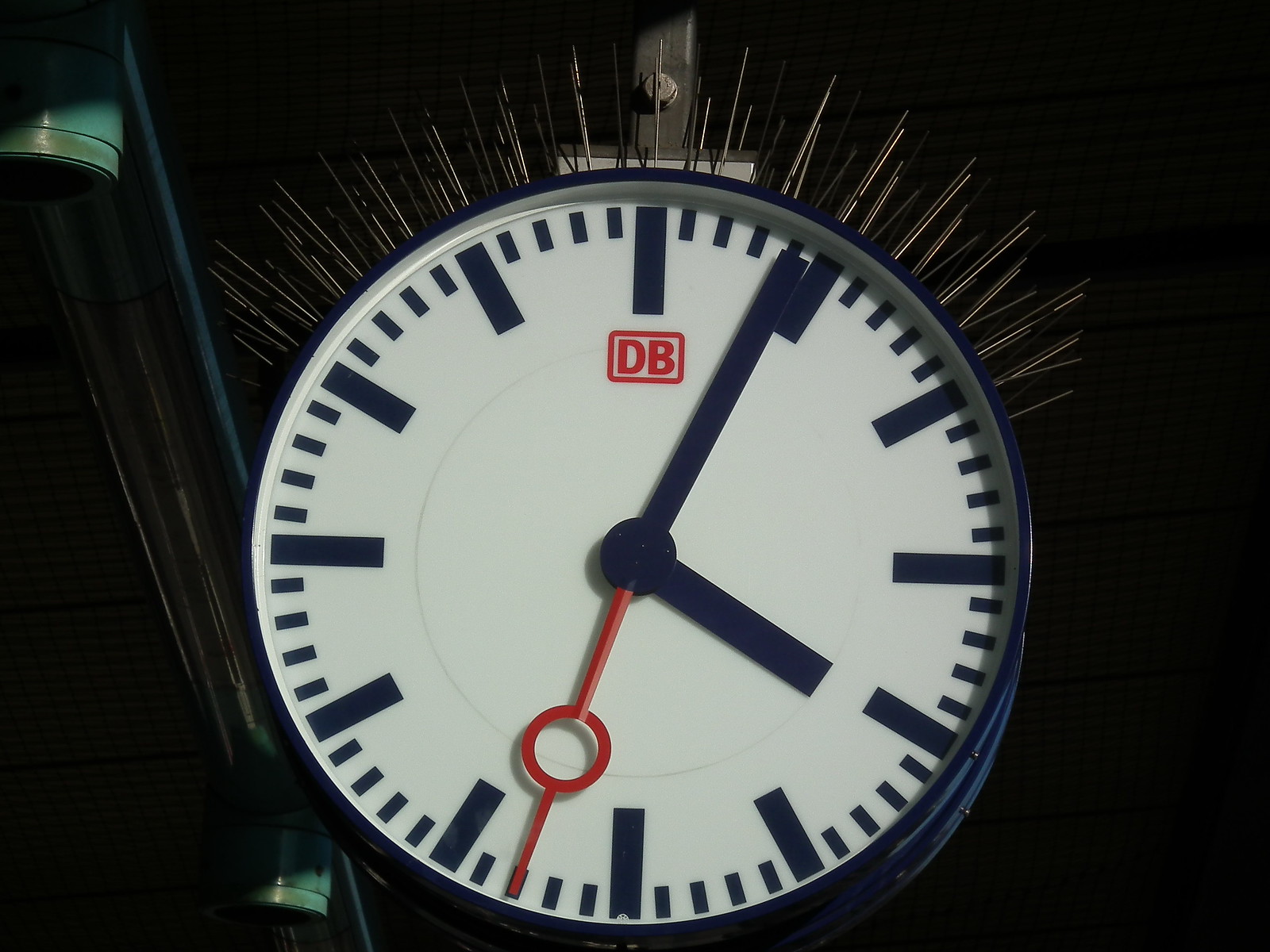This image depicts a clock with a white face set against a stark black background. The clock face is minimalist, featuring very thick lines in place of numbers to indicate the hours. The time shown is 4:04. From the top of the clock, several needle-like or nail-like protrusions stick straight upward. The clock is suspended by a metal bracket, which is visible hanging down from the top. The clock has noticeable depth, especially apparent at its bottom edge. On the left side of the image, there are some additional elements: poles and two green round objects, one positioned at the top and the other at the bottom. The function or association of these objects with the clock is unclear.